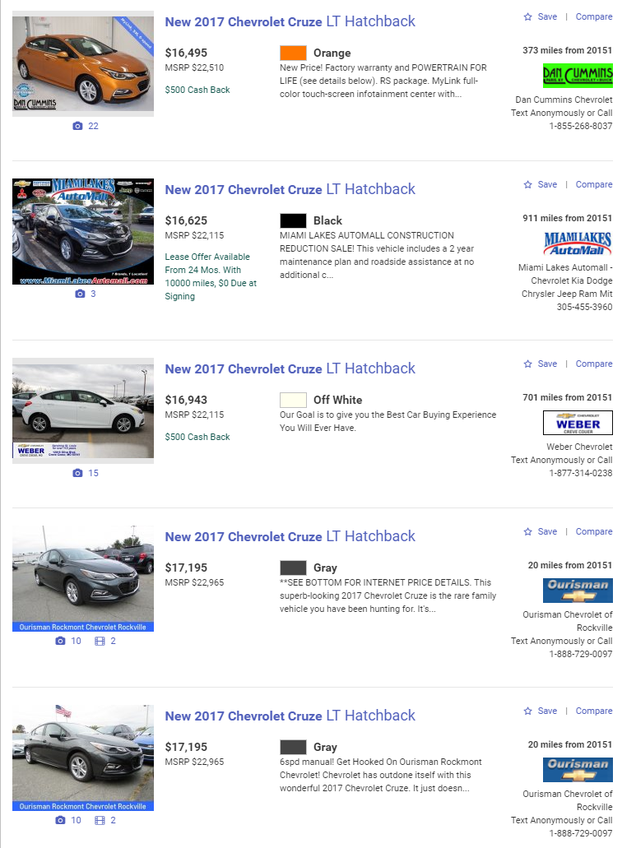This screenshot captures a detailed view of car listings from a website, presented on a clean white background with a thin, medium gray vertical line on the left edge of the page. Each car listing follows a uniform structure:

On the left, there is an angled photograph of a car. Positioned to the right of the photograph is the car's name in blue text, with a blue star icon adjacent to it. Following this is the blue text links "Save" and "Compare," separated by a thin gray line.

Directly below the car name on the left side, bold black numerals display the car's price. Beneath it, in smaller medium gray text, the term "MSRP" appears followed by another price. For the first three listings, there is a green paragraph of text underneath the MSRP information.

Next, to the right of this description, each listing features a colored rectangle, next to which appears a bold color name text. Below this, a paragraph in medium gray text provides further details about the car. 

To the right of the description, each listing indicates the distance in small black text with numbers followed by "miles from 20151."

Each listing ends with a right-justified dealership logo, under which is light gray text specifying the dealership's location and phone number.

The first listing is for an orange car, with the title "New 2017 Chevrolet Cruze LT Hatchback," and subsequent listings follow a similar format.